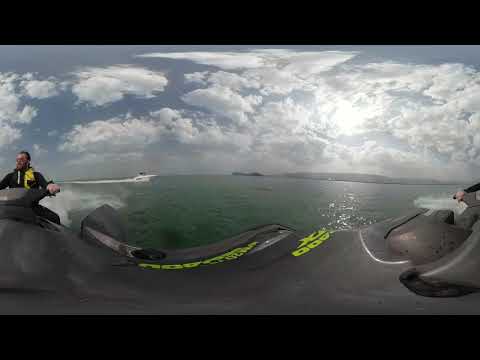This outdoor scene captures a dynamic and distorted panoramic photograph of a man riding a gray jet ski on a large greenish-blue body of water. The image is bordered by thin black bars at the top and bottom, suggesting it might be a still from a video. The sky above is dotted with numerous gray and bright clouds, with sunlight piercing through, giving the water a reflective sheen. The man, positioned on the left, has brown hair, a beard, and wears sunglasses, a long-sleeved black shirt, and a black and yellow life vest. He grips the jet ski handlebars firmly as he glides over the water. The jet ski itself is mostly black with neon green text and numbers. In the distance, a white speedboat speeds past, leaving a trail of foam. On the horizon to the right, a low-lying landmass or small mountain range is faintly visible, adding depth to the serene yet action-filled scene.